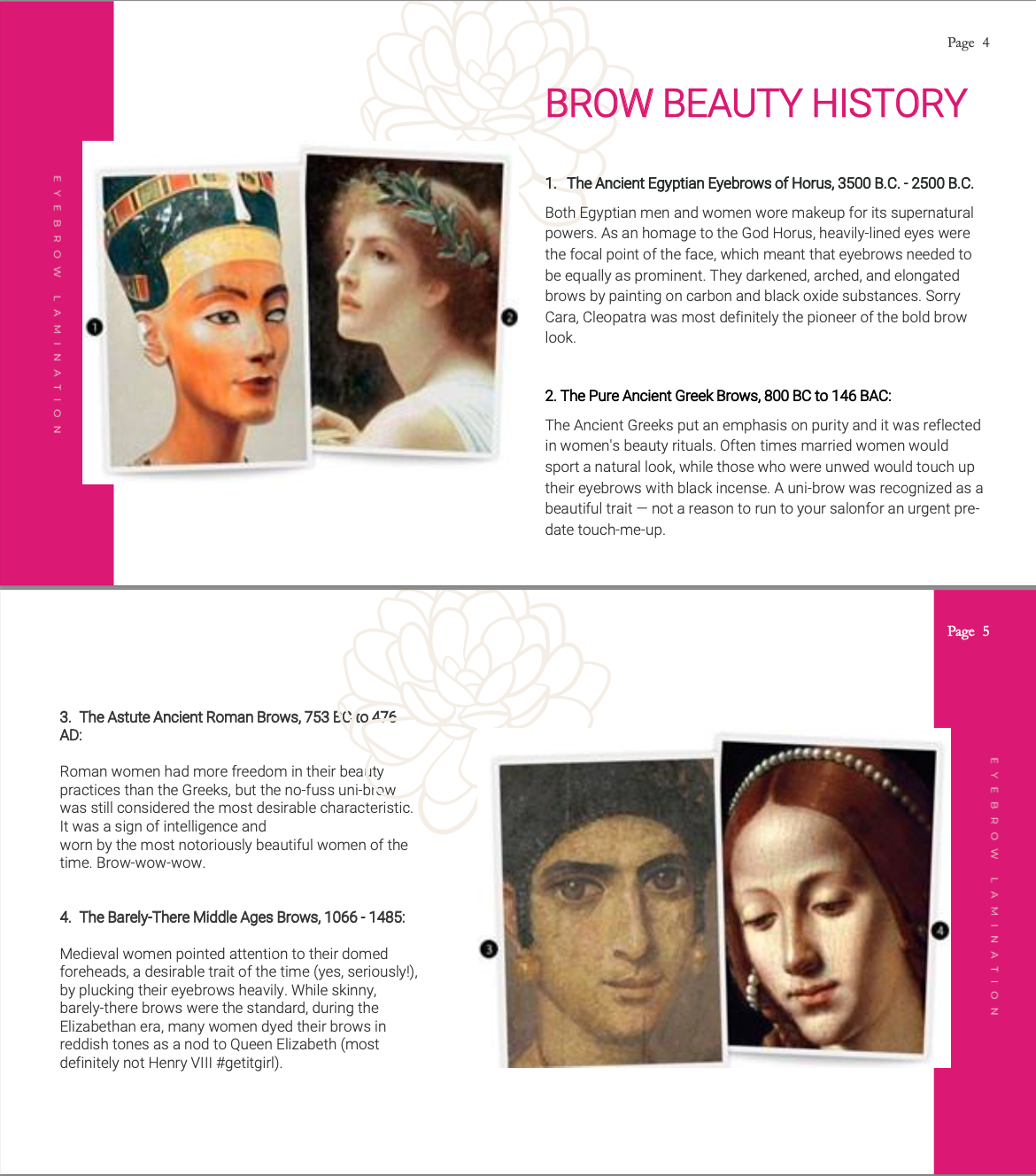The image depicts two pages from likely a magazine or encyclopedia article titled "Brow Beauty History." The upper page is designated as page 4 and features a bright pink vertical border on the left side with white print reading "eyebrow lamination." The article title "Brow Beauty History" is rendered in the same vivid pink and introduces the first historical segment titled "The Ancient Egypt Eyebrows of Horus, 3500 BC to 2500 BC." This section includes a detailed paragraph explaining how ancient Egyptians, both men and women, darkened, arched, and elongated their brows using carbon and black oxide substances to emulate the god Horus. Adjacent to this text on the left are two illustrative images: one of a pharaoh and another of a Greek goddess adorned with a leafy crown. Following is the second segment, "The Pure Ancient Greek Brows, 800 BC to 146 BC," which describes how ancient Greek women emphasized purity in their beauty rituals, sometimes even sporting unibrows as a beauty trait. The background of the text displays a brown clipart flower.

Below this, the second page, labeled page 5, mirrors the layout of the first but with the bright pink border on the right side. This page continues the historical exploration with segments titled "The Astute Ancient Roman Brows, 753 BC to 476 AD" and "The Barely There Middle Age Brows, 1066 to 1485." Each segment is accompanied by detailed paragraphs describing the era's eyebrow beauty standards and practices, and similar to the first page, features images illustrating these historical beauty trends. The recurrent motif of a light brown clipart flower is also present, adding continuity between the pages.